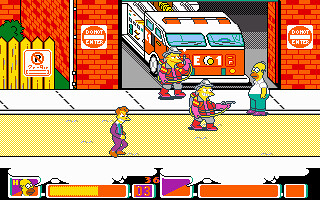This image appears to be a vibrant scene from a Simpsons video game, potentially the classic Simpsons arcade game, known for its signature bright and colorful style. The scene showcases a bustling street featuring various elements in distinct hues of white, purple, pink, red, and yellow. Central to the image is a brick fire station adorned with red and white "Do Not Enter" signs. A fire truck, predominantly red with a white top and red lettering, is stationed in the large garage opening. 

Firefighters, dressed in red jackets, gray helmets, red boots, and purple gloves, are equipped with water guns and stationed nearby. The focal point includes Homer Simpson, identifiable by his trademark white shirt, green pants, and purple boots, strolling down the street. Additionally, a man in a purple suit with yellow or orange hair is also visible, contributing to the lively scene.

The yellowish-tan road complements the white sidewalks and is bordered by a yellow picket fence adjacent to a grassy area. Health bars and a timer are displayed at the bottom of the screen, suggesting an active gameplay interface, with the timer showing “03” in red letters and a health bar partially filled with yellow. This richly detailed depiction captures the essence of the animated Springfield, blending iconic characters with vivid surroundings.